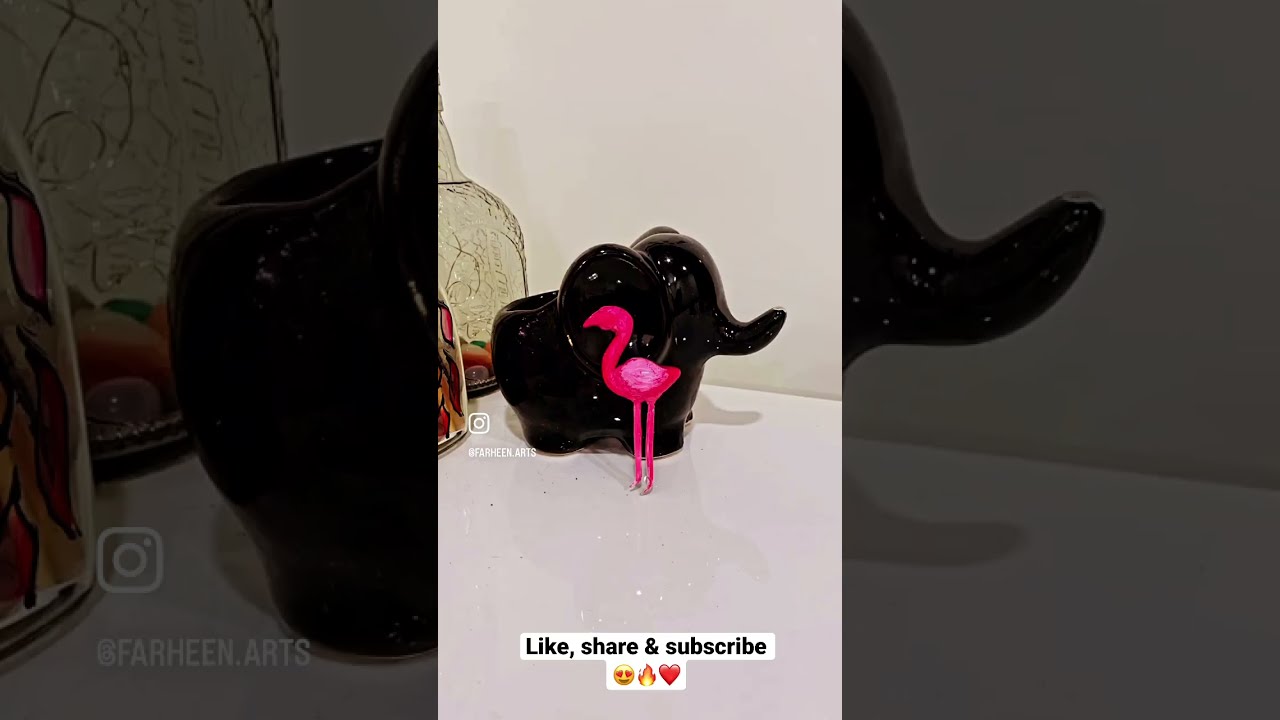The image features a detailed, multi-layered composition where a central photograph showcases two shiny sculptures—a black porcelain model of an elephant and a pink flamingo with red and pink wings. This central photograph is set against a considerably dimmer, larger background image of the same elephant sculpture, creating a layered effect. The pink flamingo, standing out in the foreground, adds a vibrant touch to the scene. Text at the bottom of the central image reads "Like, Share, and Subscribe," along with several emojis: a smiley face with heart eyes, a fire symbol, and a heart. Additionally, the bottom of the image includes an Instagram handle, @farheen.arts, and an Instagram logo, indicating that this is likely a social media post. To the right of the background image, there's a collection of indistinct glassware and an object with a design, adding extra elements to the scene.